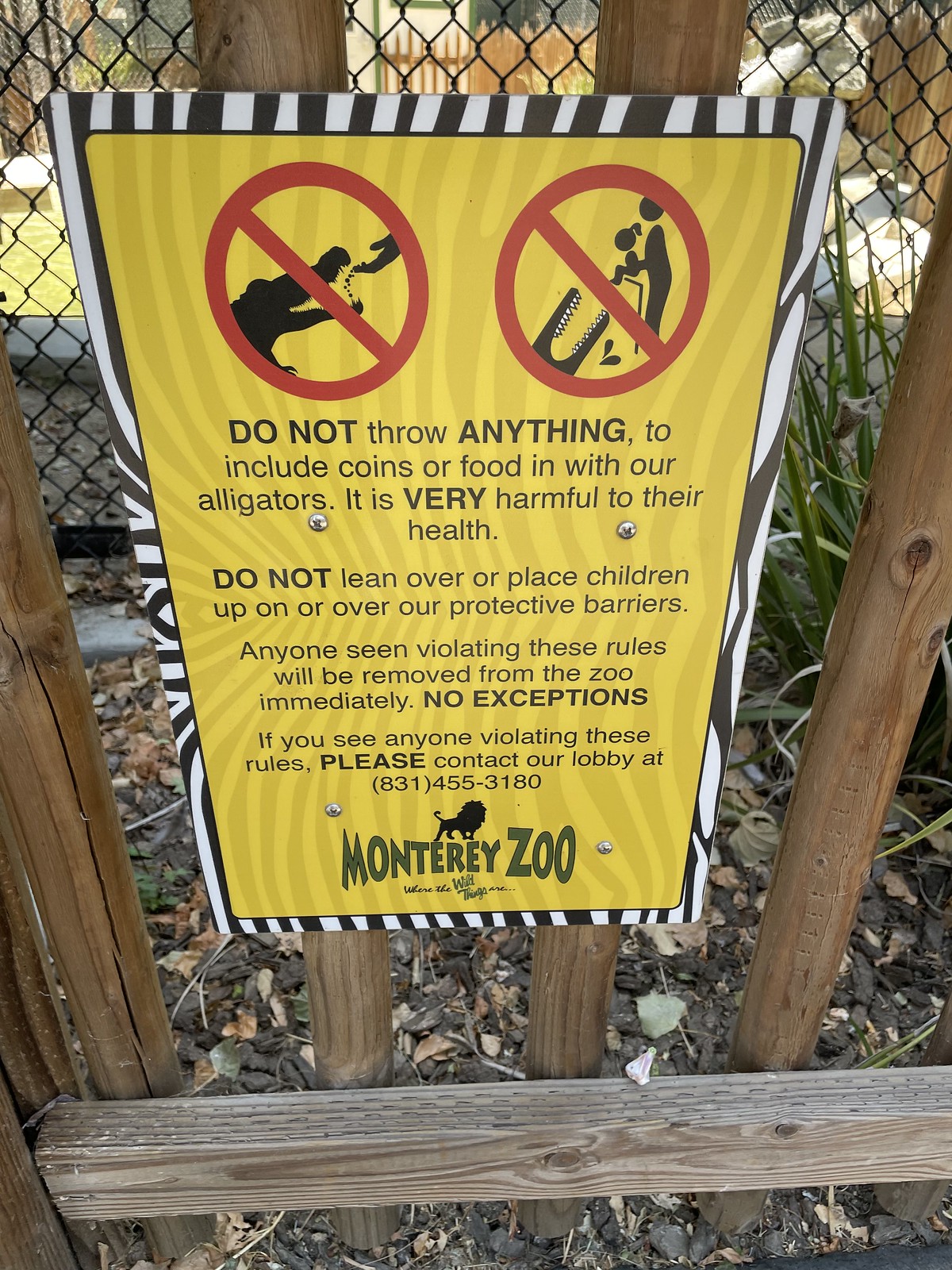The image features an informational sign prominently displayed in the center, bolted with four silver bolts to a brown wooden slotted fence. The sign is framed with a black and white zebra pattern, giving it a distinct look. The background of the main body contains a yellow and dark yellow zebra stripe design. At the top of the sign, there are two red circles with red lines cutting through them: the first depicts a shadow of an alligator with a human hand dropping crumbs into its mouth, while the second shows an adult holding a small child over an open alligator's mouth. 

The sign bears a firm warning: "Do not throw anything, including coins or food, to our alligators. It is very harmful to their health. Do not lean over or place children up on or over protective barriers. Anyone seen violating these rules will be removed from the zoo immediately. No exceptions. If you see anyone violating these rules, please contact our lobby at 831-455-3180." The sign indicates that it is by the Monterey Zoo and includes their logo at the bottom. The setting appears to be outdoors in the middle of the day, with surrounding elements including rocks, grass, and possibly hints of animals in the background.